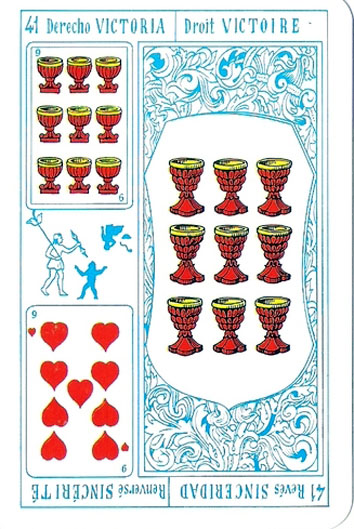This is a vintage playing card intricately adorned with detailed artwork. At the top, it features the text "Derecho Victoria," which translates to "Direct Victory." The top left corner of the card displays the number '41.' On the left side of the card, there is a red cup with a yellow top, while the right side features a yellow gauntlet. The card is predominantly decorated with nine red cups, each topped with yellow. Interwoven in the background are motifs of blue and white, lending a flowing, dynamic feel to the design. The bottom left corner houses the symbol of nine hearts. At the center, there is a character holding an indistinguishable item in their hand. The phrase "Derecho Victoria" is mirrored at the bottom of the card, completing its ornate and symmetrical layout.